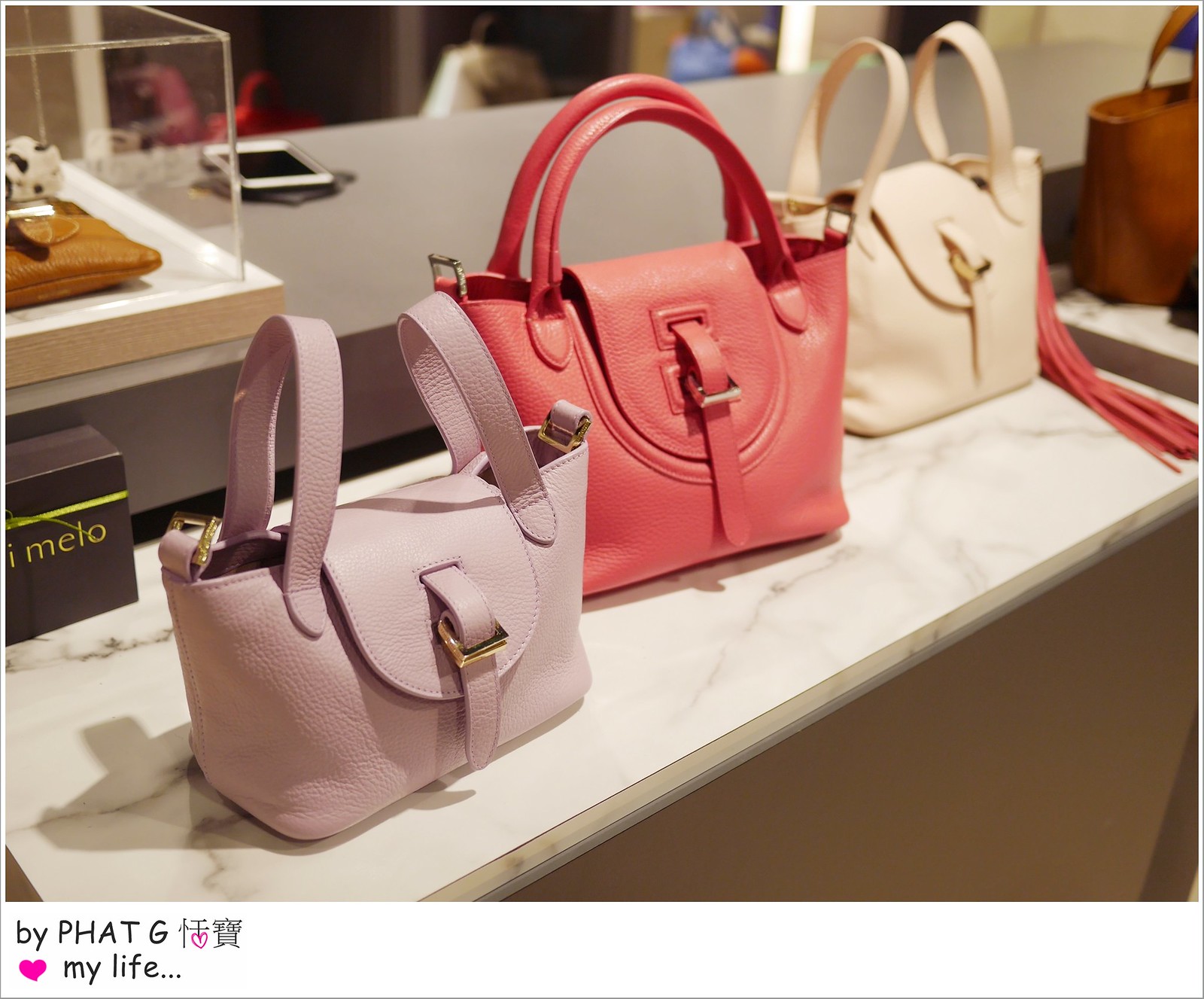This color photograph, possibly intended for a web page, showcases a luxury marble or faux-marble shelf adorned with several leather handbags. From left to right, the handbags are a dusty rose leather purse with handles pointing upward, a coral leather purse featuring a matte gold buckle at its center, and an off-white or cream leather purse with an attached coral-colored scarf or fringe. Partially visible on the far right is a brown leather handbag. Behind the handbags, a plexiglass cube displays an unspecified item, while a cardboard box with gold lettering spelling "Mello" sits nearby. The snapshot includes a signature at the bottom, resembling a Polaroid photo caption, which reads: "by Phat G," accompanied by Asian ideograms, a heart symbol, and the inscription "My life..."